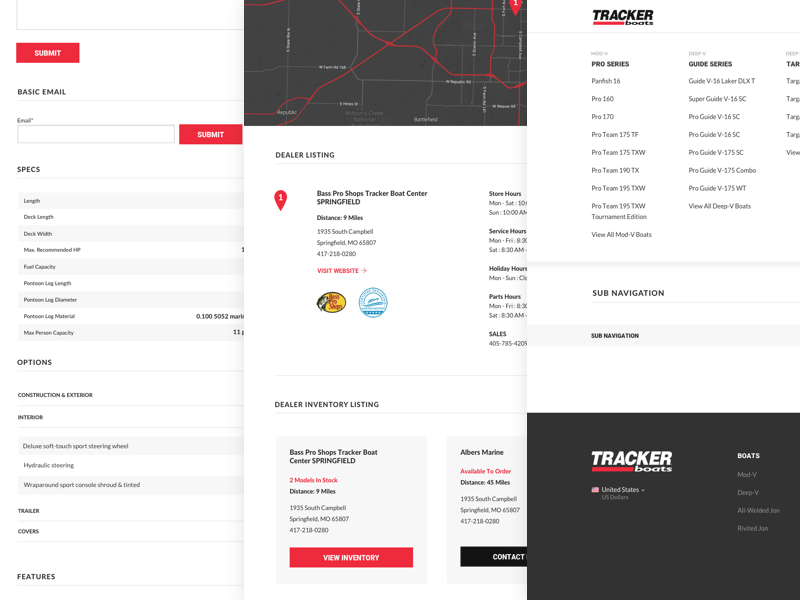This image is a composite of three cropped screenshots from the same webpage, likely from a desktop website, arranged side-by-side. Each screenshot appears in a format resembling that of a mobile device. 

On the left side of the composite, the first screenshot features a white background and begins with a red "Submit" button followed by a text box for email input. Below it is another red "Submit" button and a section titled "Specs." Along the left margin, there are several categories listed, such as "Length," "Deck Length," "Deck Width," and "Fuel Capacity," though the specific values are not visible due to cropping.

The middle screenshot shows a dark gray map that provides directions to a dealership, specifically to a Bass Pro Shops Tracker Boat Center. The map highlights the route in red.

The final screenshot on the right displays the footer of the website, which contains links to various boat-related pages. The text in the footer is small and somewhat difficult to read but includes the label "Tracker Boats."